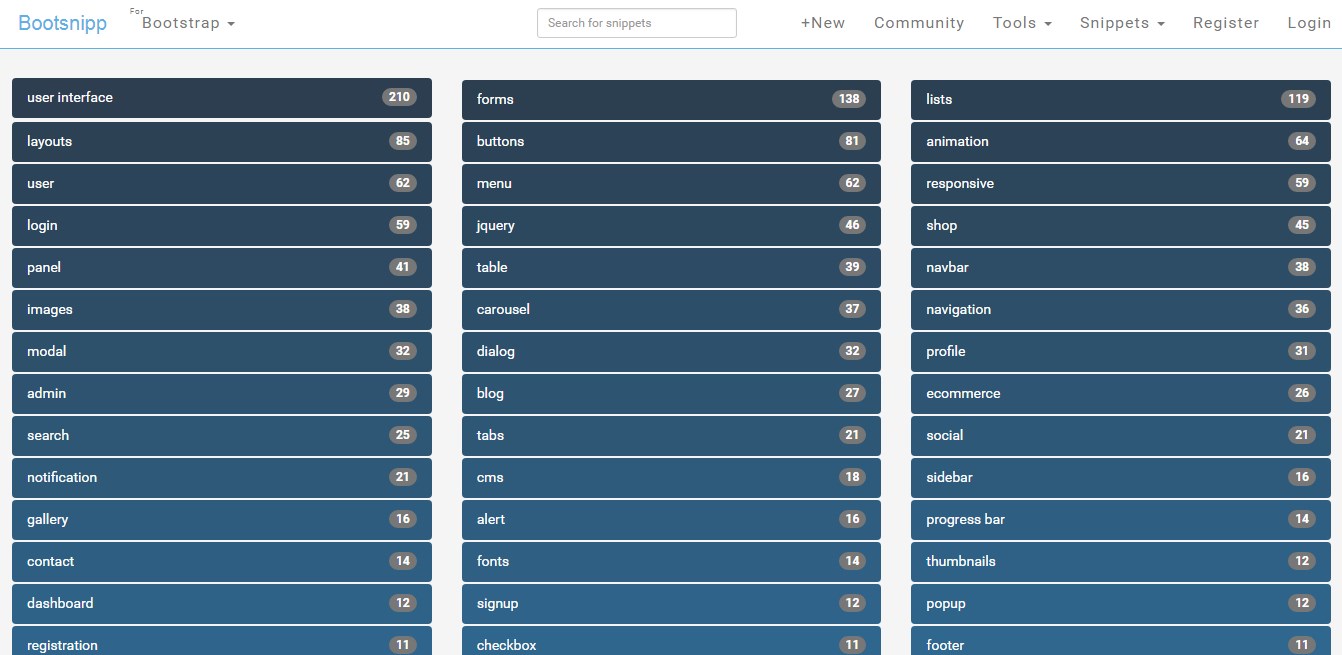The website for BOOTSNIPP (spelled B-O-O-T-S-N-I-P-P) features the logo prominently in the upper left-hand corner. To the right of the logo, there's a drop-down menu labeled BOOTSTRAP. Occupying the top header of the page, there’s a search box positioned towards the left, followed by links for "New Community Tools," "Snippets" (each with its own drop-down menu), and options for "Register" and "Log In" aligned towards the right.

Below the header, the page's body comprises several long rectangular boxes in blue with white text. The layout is organized into three sections, each containing approximately 10 rows of these boxes stacked from top to bottom. 

At the very top left of these sections, the first box is labeled "User Interface" with the number "210" to its right. Adjacent to it are boxes labeled "Forms" with "128" next to it, and "Lists" with "119."

In the bottom row of these sections, starting from the left, the first box is labeled "Registration" with "11" to the right. Following that, there is a box labeled "Checkbox" with "11" next to it, and finally, on the bottom right, a box labeled "Footer" also with "11" on its right side.